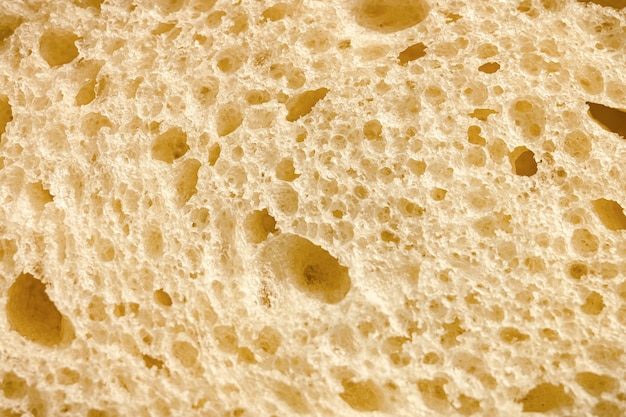This image is a close-up of a piece of flatbread, possibly naan, tortilla, or matzah. The bread features a beige to a very light tan hue with a slight yellow tint, and is dotted with numerous pockmarks resembling craters. These air pockets vary significantly in size and depth—some are quite small and shallow, while others are large and deep, creating a textured surface. The larger, darker pockets have jagged, oval shapes, whereas the smaller ones are dispersed more randomly. The light catches the higher, craggy areas, creating shadows in the deeper crevices and showcasing the rough, grainy texture of the bread. Prominent clusters of air pockets are noted throughout the image, including a small one in the top left, a large one in the top right, and a mix of variously sized pockets in the center and bottom sections. The overall appearance conveys a tightly crumbed bread with detailed shadowing and highlights accentuating its baked intricacies.